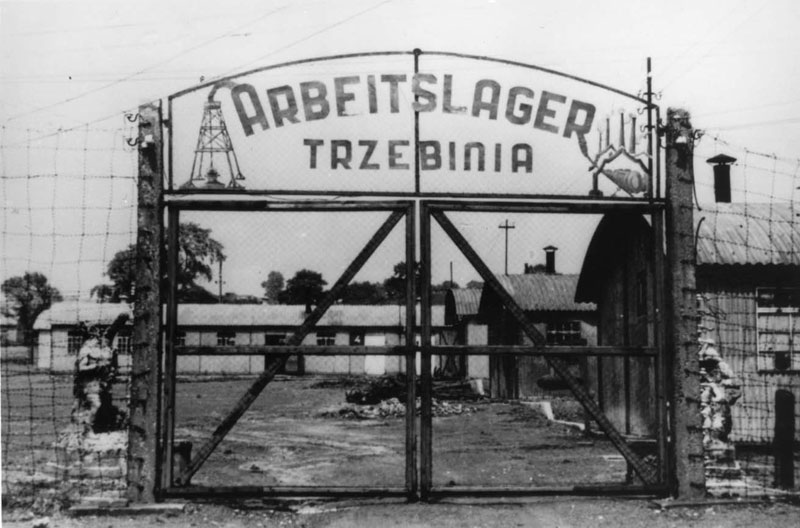In this black and white photograph, a stark, old image captures the entrance to what appears to be a concentration camp. The centerpiece is a dark metal gate, flanked by areas of mesh wire. Just above the gate is a white sign with bold, dark letters that read "Arbeitslager" and "Trzebinia." Artwork adorns either side of the sign, featuring what looks like an oil derrick on the left and a chimney or smokestacks on the right. Beyond the gate, the ground appears to be dirt, and the background reveals four small, cabin-like houses with corrugated metal roofs and dark smokestacks. Electrical poles dot the landscape further back, leading to a backdrop of trees under a gray sky.